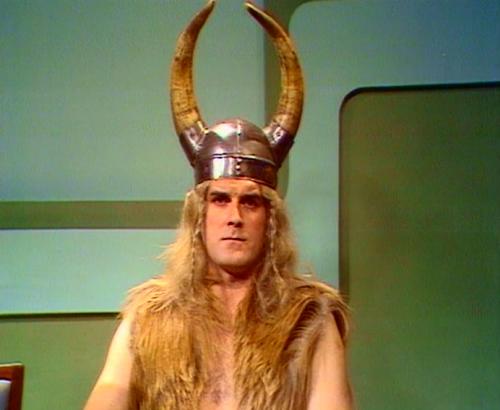The photograph, which has a grainy, older quality to it, depicts a man with a strong, square jaw and long blonde hair that reaches just below his shoulders. The front sections of his hair are styled into braids on both sides. He is donning a Viking-style helmet made of metal, featuring two slightly yellowed horns that point inward at the top. The man is facing directly towards the camera with an intense gaze. He is dressed in a fur vest with long, blonde fur, leaving his arms and chest exposed. Behind him, the background consists of textured panels in varying shades of green—a dark green dominates the bottom and the right side, while the top left features a much lighter green. An almost S-shaped light green line runs through the background. In the lower left corner of the image, there is a small object that appears to be the top corner of a wooden, padded chair. The setting seems to be an older building with a 60s aesthetic, adding to the photograph’s vintage feel.